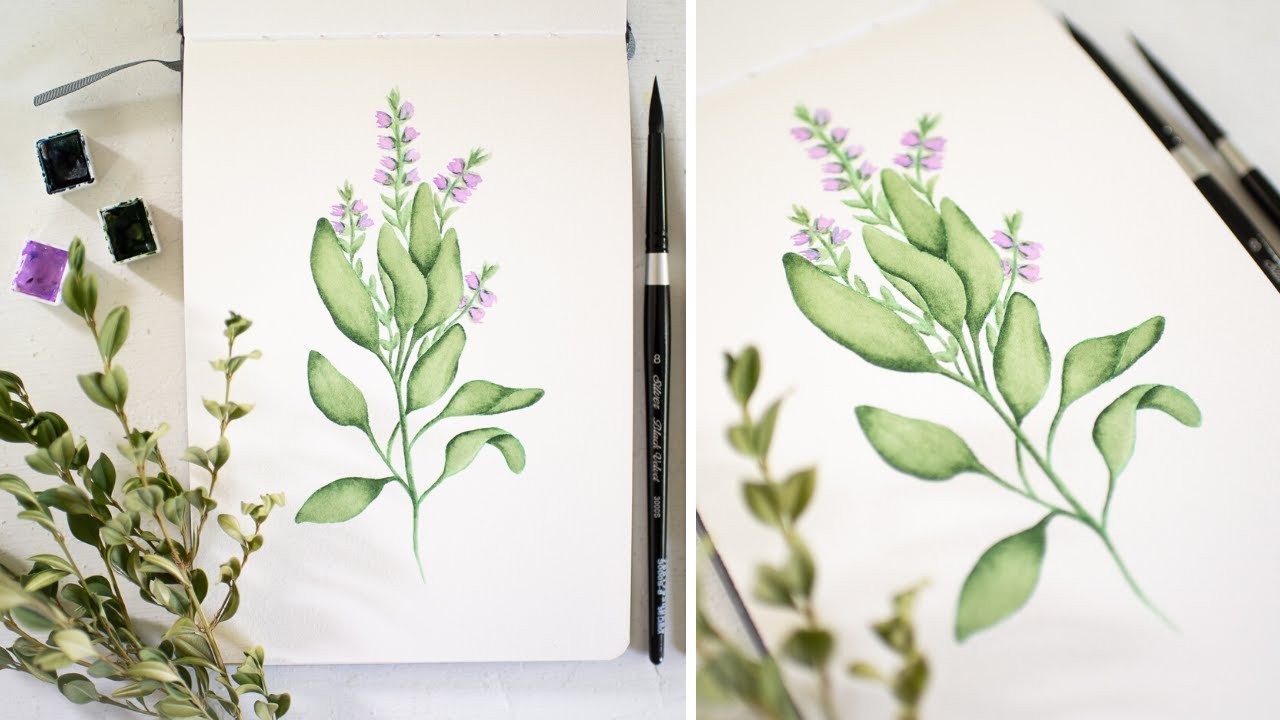The image showcases a dual-angle view of a calligraphy set and a watercolor painting. On the left, a painting on a drawing pad displays a botanical subject: green leaves with darker outlines extending from a thin stalk, crowned with clusters of purple flower tips. The live reference plant, with similar green leaves but dried and missing the purple flowers, is positioned to the left of the canvas. Adjacent to the pad is a black brush labeled 'Size 8,' alongside three paint containers—two black and one purple. On the right, a closer, diagonal view reveals finer details of the watercolor artwork, emphasizing the meticulous rendering of the green foliage and delicate purple blossoms, echoing the natural subject nearby.